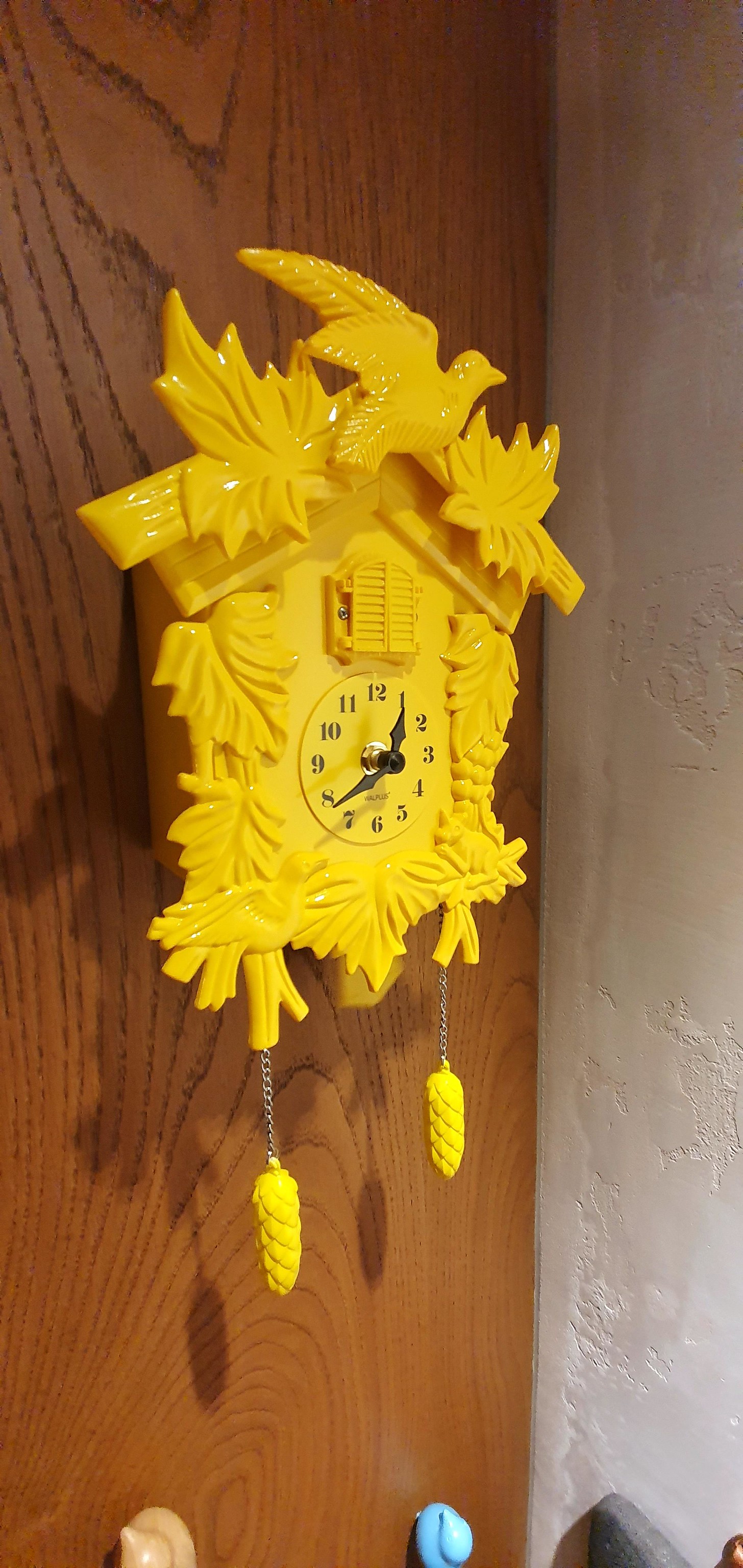This image showcases an angled view of a vibrant yellow plastic cuckoo clock hanging on a wooden wall, located near the corner where the wooden surface meets a white painted concrete wall. The clock is designed with a small, rounded, yellow door below the roof, where the cuckoo bird emerges to announce the time. The door features horizontal lines imitating wood slats. Above the door sits a bird surrounded by two large, angled leaves—one pointing left and the other right. 

The clock's face is relatively small, featuring black numbers and black metal minute and hour hands, indicating the time at 1:40. The border around the clock face is adorned with ornate leaves, enhancing its detailed design. Additionally, two long acorn-shaped pendulums dangle from chains on either side of the clock. Completing the intricate design, there are two more birds perched—one in the bottom left corner and the other in the bottom right corner of the clock.